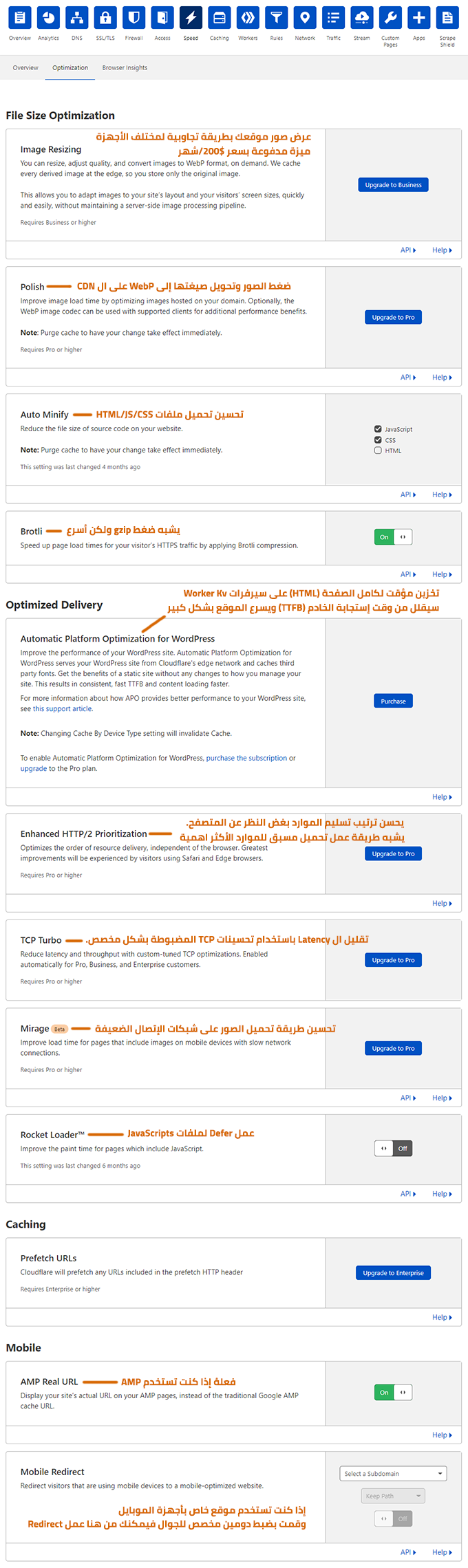The image appears to be a screenshot of a software interface from a computer program, likely related to website optimization. At the top, a horizontal toolbar features a variety of icons, predominantly blue with white symbols, each accompanied by descriptive text. Among these, an icon with a darker blue background labeled "Speed," illustrated with a lightning bolt, stands out. 

Beneath this toolbar, three main categories are listed: Overview, Optimization, and Browsing Insights. The "Optimization" tab is currently active, indicated by an underline. Within this tab, several rectangular modules with distinct functionalities are displayed, including:

1. **Image Resizing**
2. **Polish**
3. **Auto Minify**
4. **Brotli**
5. **Optimize Delivery**
6. **Automatic Platform Optimization for WordPress:** This option includes a blue button labeled "Purchase."
7. **Enhanced HTTP/2.0 Prioritization:** Accompanied by a prompt to "Upgrade to Pro."
8. **TCP Turbo**
9. **Mirage**
10. **Rocket Loader**
11. **Mobile**
12. **Mobile Redirect**

Each module appears to offer specific enhancements and settings to improve website speed and performance. The "Purchase" and "Upgrade to Pro" options suggest additional features may be available in a premium version of the software.